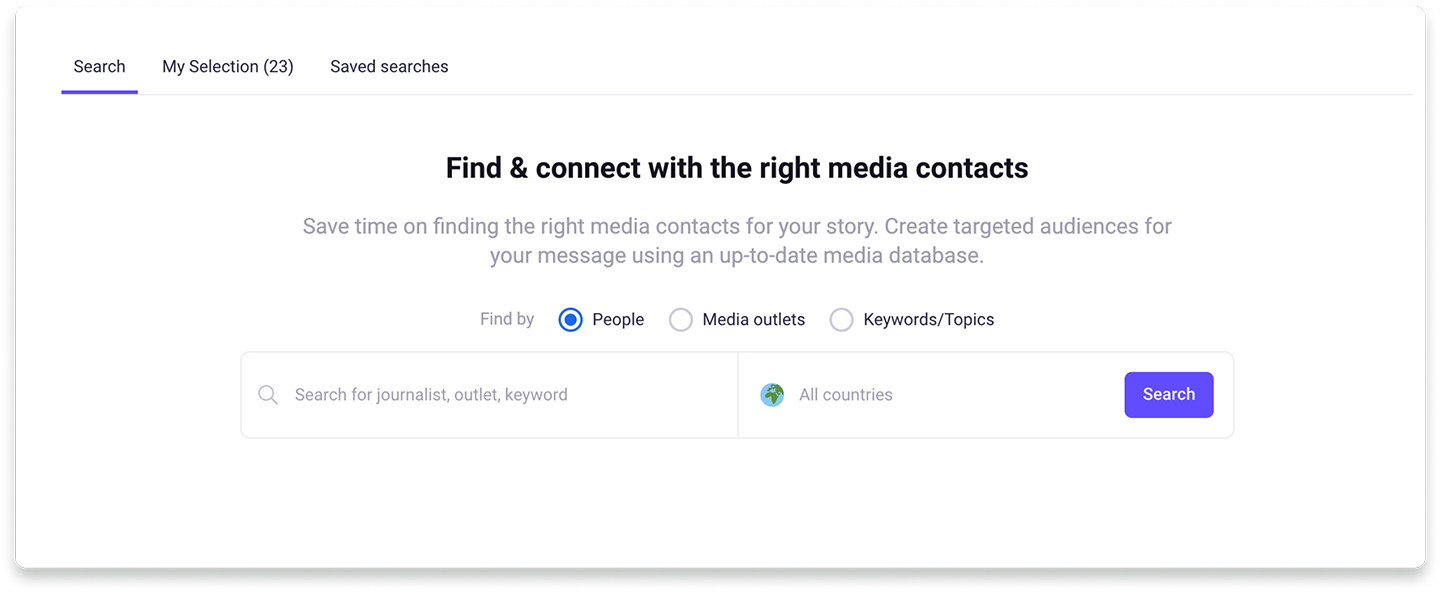The image features a user interface set against a clean, white background. Central to the interface is a search bar adorned with an icon of a magnifying glass. Adjacent to the search bar, a blue rectangle button labeled "Search" in white text is easily noticeable. 

Above the search bar, there is a selection dropdown with the text "Save Searches" and an option denoted by the number "23" in parentheses. Below the search bar, there are multiple options to refine the search including "Find and connect with the right media contacts," "Save time on finding the right media contacts for your story," and "Create targeted audiences for your messages using an up-to-date media database."

Three circular radio dial buttons are positioned below these options, each allowing the user to filter results by specific criteria: the first one, labeled "People," is shaded to indicate it is active; the second, labeled "Media Outlets"; and the third, labeled "Keywords & Topics."

Beneath this, a section is devoted to selecting countries, represented visually by a tiny globe icon featuring green land and darker green waters. All these elements are designed to facilitate the user's search for journalists, media outlets, or specific keywords across various countries.